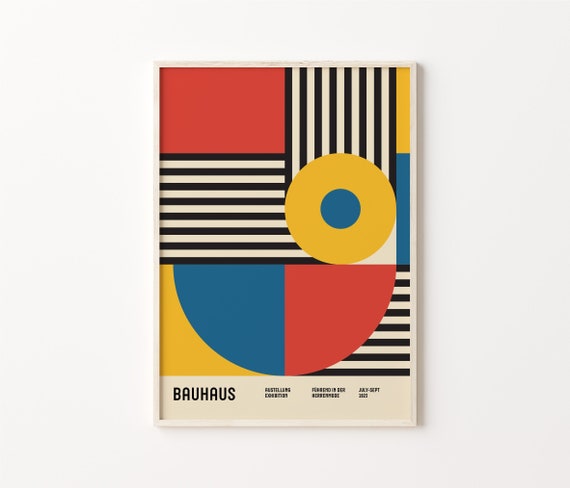The artwork displayed in a white frame is a modern abstraction deeply rooted in the Bauhaus aesthetic. Measuring approximately 16x12 inches, the geometric painting is divided into various distinctive sections, each brimming with vibrant and contrasting colors. At the top left, a bold red square commands attention, juxtaposed by a thin vertical yellow rectangle on the top right. Below the red square, black and white stripes create a dynamic contrast, and these stripes extend to the middle of the piece, originating from a yellow circle with a smaller blue circle inside it, reminiscent of a vinyl record. The bottom section features a semi-circle composed of blue and red segments interspersed with more black and white stripes. The entire composition rests atop a white bar at the bottom, where the word "Bauhaus" is inscribed in black text, accompanied by three additional unreadable sections of text. This detailed arrangement creates a visually engaging and thought-provoking representation of the Bauhaus movement's principles.